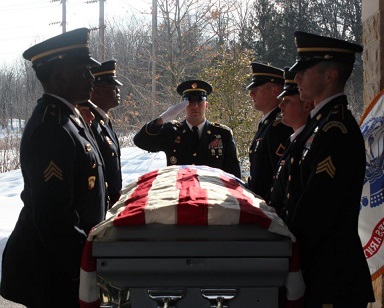This photograph captures a solemn winter scene at a military funeral procession. In the center, a brown casket adorned with silver handles is meticulously draped with a neatly folded American flag. Three soldiers in formal navy blue uniforms with matching caps and white dress shirts line each side of the casket, their gloved hands gripping it securely. A seventh soldier stands at the head of the casket, saluting with his right hand in a white glove. The backdrop features a gray sky with the sun breaking through, illuminating snowy terrain, indicating a cold winter setting. To the right, partially visible, is another flag, likely a military division banner. Light poles and leafless trees in the background add to the outdoor, wintry atmosphere of the ceremony.